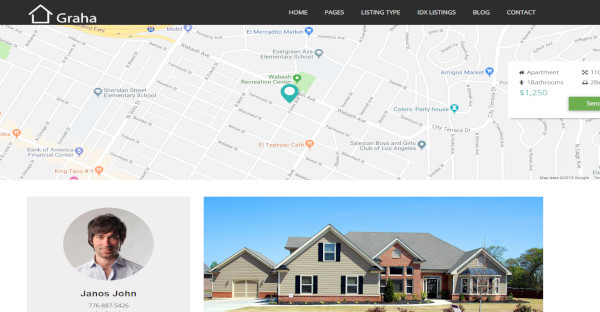The image features a black navigation bar at the top. On the left side of the bar, there is an icon of a house with the text "Graha" next to it. Moving towards the right, the bar includes links labeled "Home," "Pages," "Listings," "Type," and "Blog." Finally, on the far right, there is a "Contact" link.

Below this navigation bar, a map is displayed, dotted with push pins marking various locations. A pop-up box on the map indicates a specific point with the number "1250" and a green button nearby.

Beneath the map is a light gray section. On the left side of this section, there is a gray circle containing an image of a man smiling directly at the camera. He has black hair, a stubble, and is wearing a light-colored shirt with a collar. His contact information is listed as "John O'John, 776-887-5426."

To the right of the man's photo is a small, well-maintained picture of a house with an A-frame roof, surrounded by a manicured lawn and a bright blue sky.